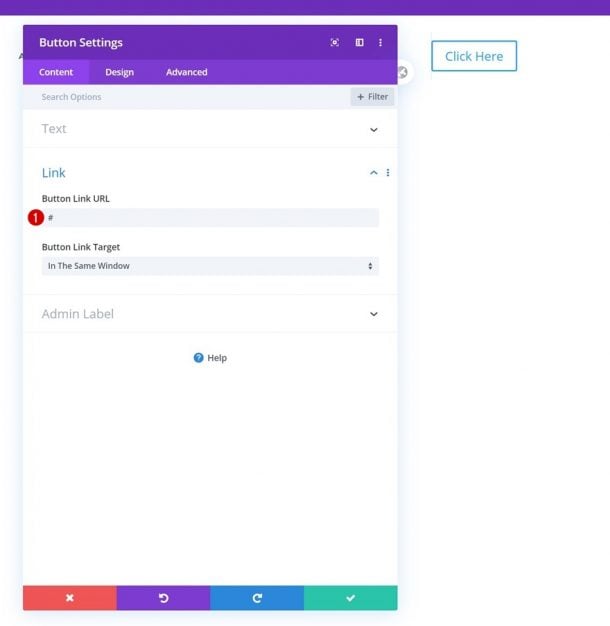The image depicts a screen from a software application, most likely viewed on a PC or laptop. At the very top, a dark purple strip spans the width of the screen but contains no visible elements. 

Towards the far right of the background, there is a blue box with the text "Click Here" written in it. In the foreground, a window is open with the heading "Button Settings" displayed in white text against a purple strip background. Directly below "Button Settings," there are three tab options: "Content," "Design," and "Advanced," also in white text on a purple background.

Beneath these tabs, there is a search option with the prompt to "Select a Filter" and a button labeled "+ Filter." Below this, a text box is present—a dropdown menu where additional options can be selected. Following that, the word "Link" is written in blue text, with a field labeled "Button Link URL" beside it. To the left of this input field, a red circle with a white "1" indicates a notification or an alert.

Further down, the label "Button Link Target" specifies that the link will open in the same window. Another dropdown menu labeled "Admin Label" appears in light gray. Below this, there is a blue circle with a white question mark next to it, accompanied by the word "Help."

At the very bottom of the window, there are four action tabs: 
1. A red tab with a white cross, presumably to close the window.
2. A purple tab with a circular arrow pointing left, likely a back button.
3. A blue tab with a circular arrow pointing right, probably a forward button.
4. A light greenish-blue tab with a white tick mark, presumably to confirm or save any changes made.